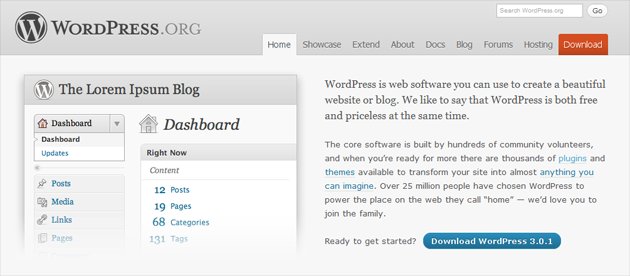The screenshot showcases the dashboard of a WordPress.com website, specifically for a blog labeled "L-O-R-E-M-I-P-S-U-M." On the left side, the detailed dashboard menu includes options such as Posts, Media, Links, Pages, and Comments. The "Right Now" section indicates the blog's current statistics: 12 posts, 19 pages, 68 categories, and 131 tags. To the right, there is a comprehensive description of WordPress, highlighting it as powerful web software for creating websites or blogs, which is both free and invaluable. It underscores the extensive support from a large community, alongside numerous plugins and themes available for customization. Additionally, it notes that over 25 million people use WordPress. At the bottom, a prominent blue button labeled "Download WordPress" urges users to download WordPress 3.1.1, reinforcing the call to action.